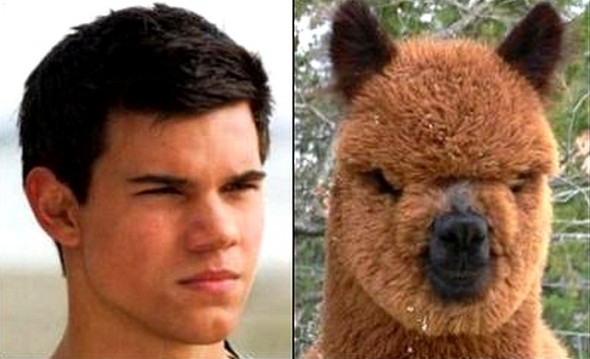The image consists of two head shots positioned side by side. On the left is a close-up of a light-skinned male with dark brown hair and eyebrows. He is squinting his eyes, as if looking into the sun, which gives him a serious expression. The background behind him is bright and slightly fuzzy, with a sand-colored lower half suggesting a beach-like setting. 

On the right is a close-up of a furry brown animal, likely an alpaca or lemur. The animal also has dark brown ears that stick up and a prominent dark black nose. It is similarly squinting with a serious expression, mirroring the human's face. The background features green trees. The juxtaposition creates a humorous comparison, emphasizing the striking resemblance between the man's intense squint and the animal's similar expression.